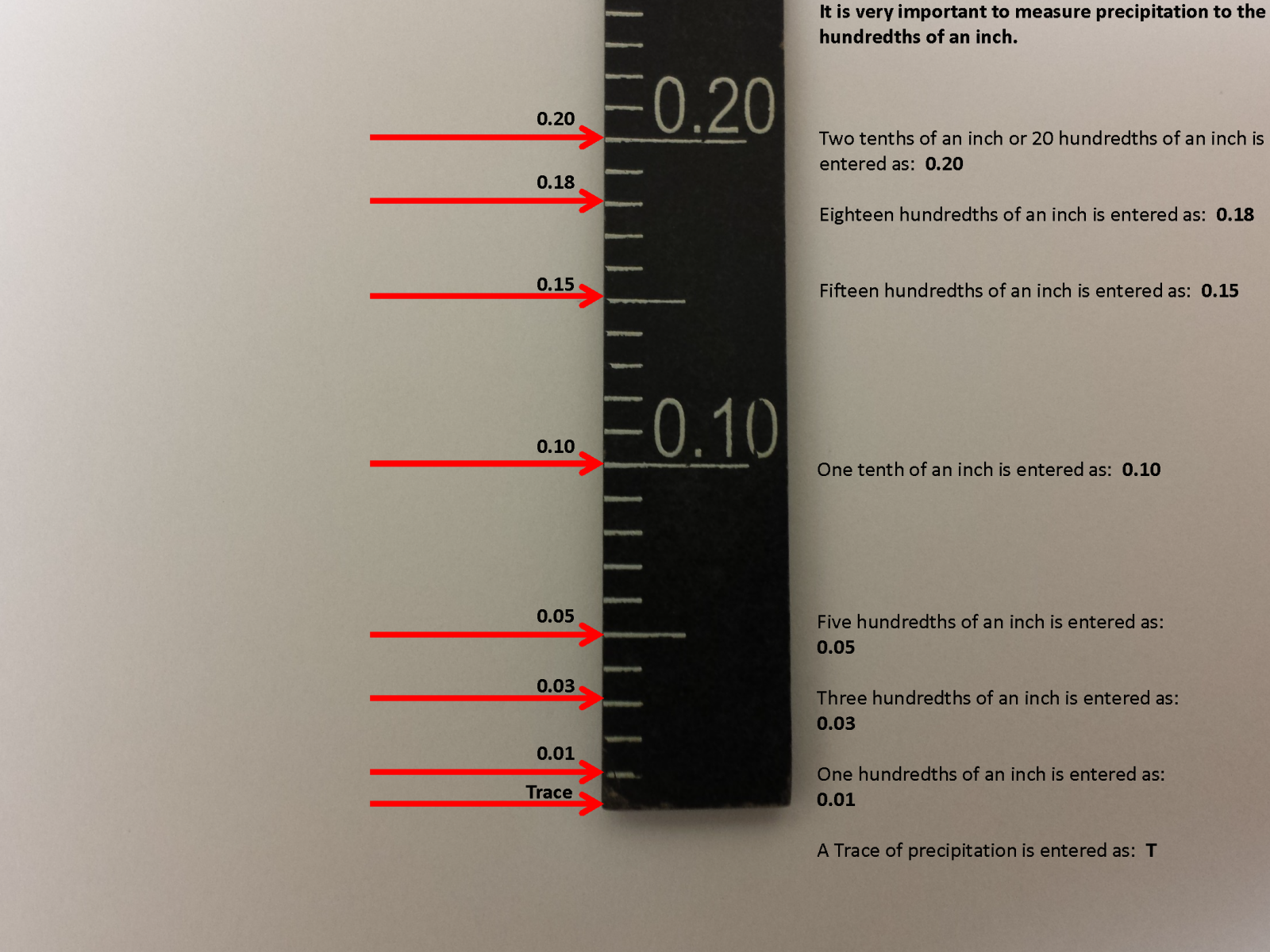The image displays a black ruler positioned vertically against a white piece of paper with black typed text explaining its components. The ruler features sequential white lines and numerical markings in hundredths of an inch, including 0.01, 0.03, 0.05, 0.10, 0.15, 0.18, and 0.20. Red arrows on its left side align with these markings, and each is labeled accordingly: "trace" (T), 0.01, 0.03, 0.05, 0.10, 0.15, 0.18, and 0.20. The right side of the ruler contains detailed text explaining that a trace of precipitation is denoted as T, and measurements progress in increments, reaching up to 0.20. The description emphasizes the importance of measuring precipitation to the hundredth of an inch.